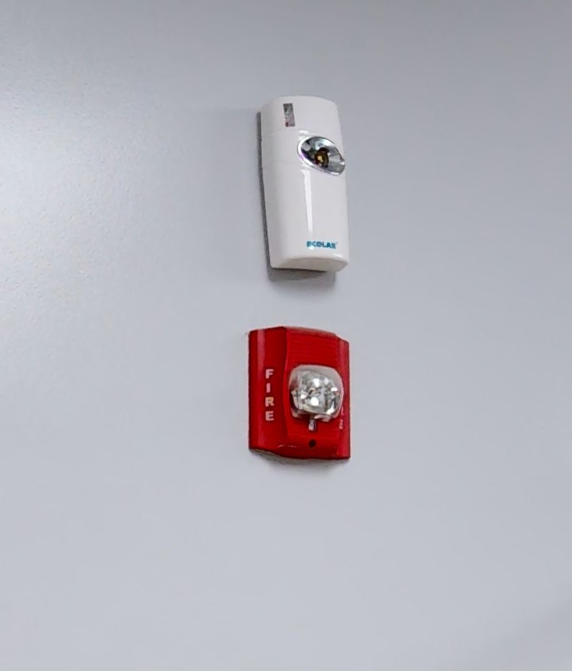The image features two distinct alarm systems mounted on a plain white wall. The lower device is a typical red fire alarm box with the word "FIRE" prominently displayed in white text on both its vertical sides. This red fire alarm is equipped with a white strobe light on its front, presumably designed to flash in emergency situations. Above it, the second system is a slightly larger, white rectangular unit labeled "Ecolab" in blue text at the bottom. This white device has a silver circular depression on its front, housing what appears to be a light, possibly a strobe light, which is either red or orange in color. Both alarms serve distinct purposes, with the lower red box clearly identified as a fire alarm and the upper white unit potentially serving a different but related safety function, such as a carbon monoxide detector.